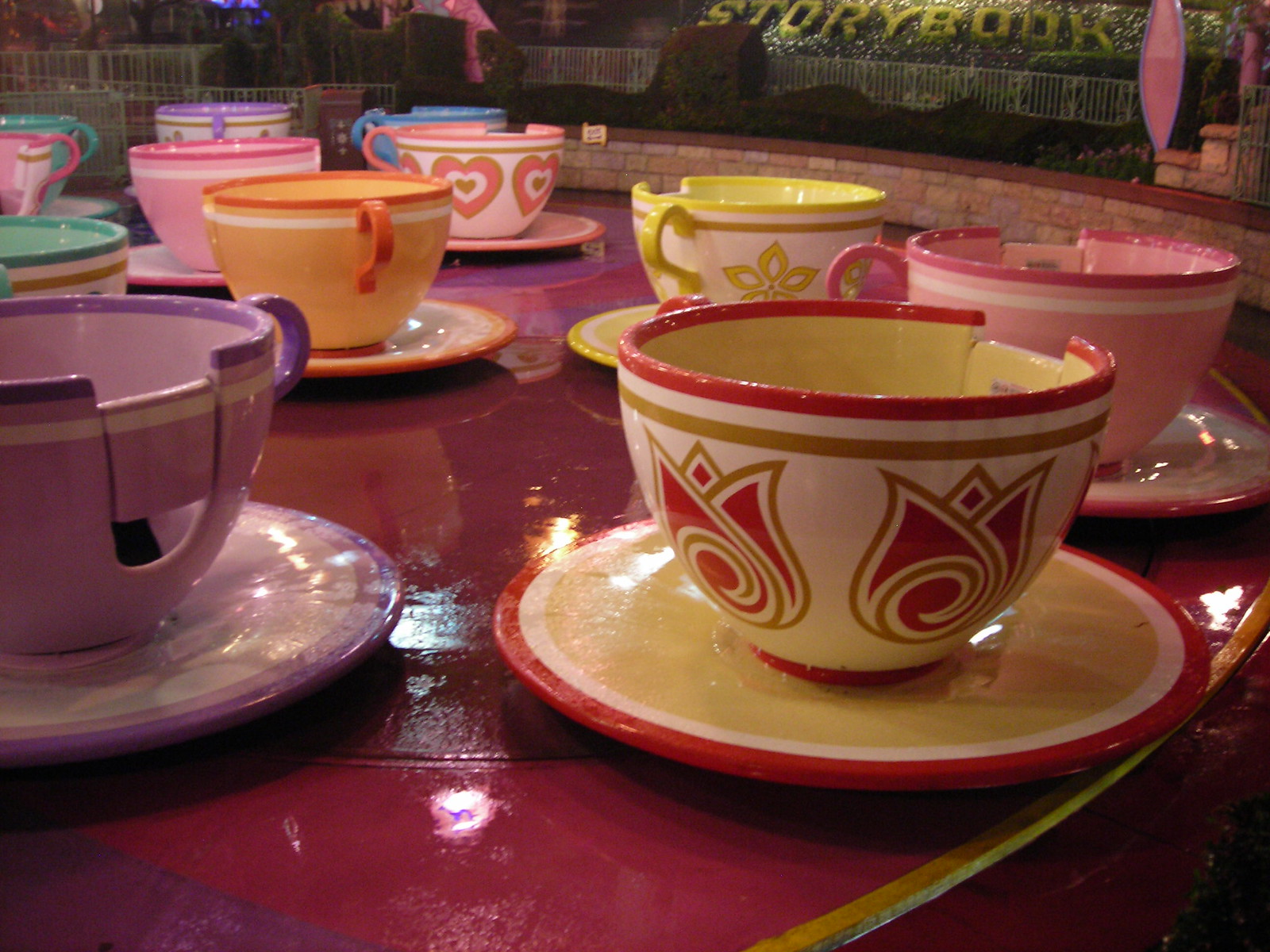The image captures a vibrant and colorful scene featuring an array of teacups and saucers set on a red table with a purple trim. Each teacup, uniquely designed in bright colors including purple, orange, pink, yellow, blue, and teal, sits on a matching saucer. Notably, these teacups have a peculiar feature: a small door-like opening that can be expanded, making them more like amusement park ride seats than actual teacups for drinking. The teacups are shiny and porcelain-looking, reflecting overhead lights, contributing to the overall vividness of the picture. In the background, the word "STORYBOOK" is meticulously crafted in green text that appears to be made out of bushes, further supporting the idea of an amusement park theme. A white fence surrounds the setting, suggesting it's an area where visitors might line up for a ride. The scene is whimsical and enchanting, brimming with charm and vivid details.